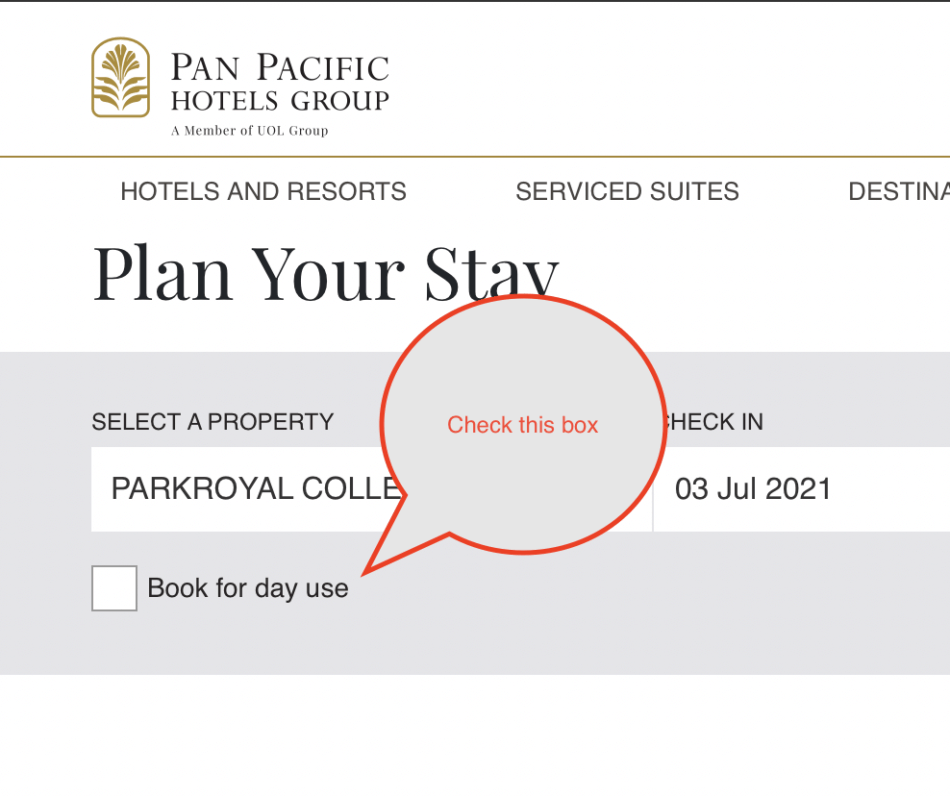The image features a rectangular layout. At the very top, there is a solid black line, immediately below which sits a gold emblem resembling a stylized leaf with three smaller leaves extending symmetrically from each side. The emblem is somewhat reminiscent of the NBC peacock, but rendered in gold.

Beneath the emblem, the text "Pan Pacific Hotel Group" is prominently displayed. Below this, another black line horizontally bisects the rectangle. Underneath the line, the text reads: "Hotels and Resorts, Service Suites, and Destinations," although the word "Destinations" is partially cut off.

Further down the rectangle, the phrase "Plan Your Stay" is written in large black letters. This is followed by a gray rectangle, within which is a smaller white rectangle positioned partway down.

Overlapping both the gray and white sections is a speech bubble with the text, "Check this box." Within the gray portion of the rectangle, the text reads: "Select a Property, Check In." The white section contains the details: "Park Royal, COLLE, 03 July 2021." Below this, a small white box says, "Book for Day Use."